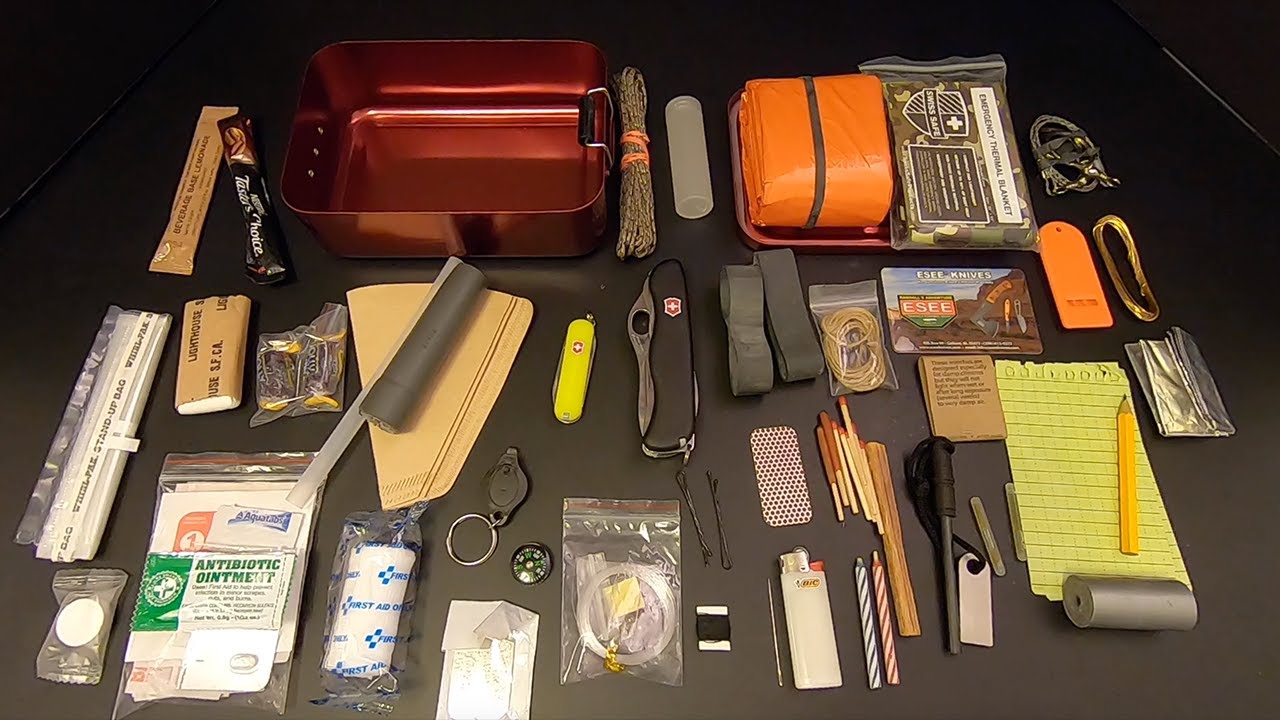This detailed color photograph showcases the diverse contents of a survival kit, all neatly arranged on a brown table. In the upper left corner, there's a distinctive red tin that stands empty. Next to it, a small rope is carefully tied up. Key survival tools include an orange tarp and a notebook accompanied by a pencil. Fire-starting essentials are well-represented, featuring flint, matches, a Bic lighter, and two candles. The kit also contains two knives: a survival knife and a smaller Swiss Army knife. Fishing needs are covered with fishing wire and a hook. Additional essential items include a small keychain light, a versatile battery, comprehensive first aid supplies, a coil of copper wire, and a folded piece of aluminum foil. The layout also features other pragmatic items like powdered drinks, twist ties, a compass, a match striker, straps, twine, duct tape, and an emergency camping blanket. The orderly arrangement and variety of items emphasize the thoroughness and preparedness inherent in this survival kit.